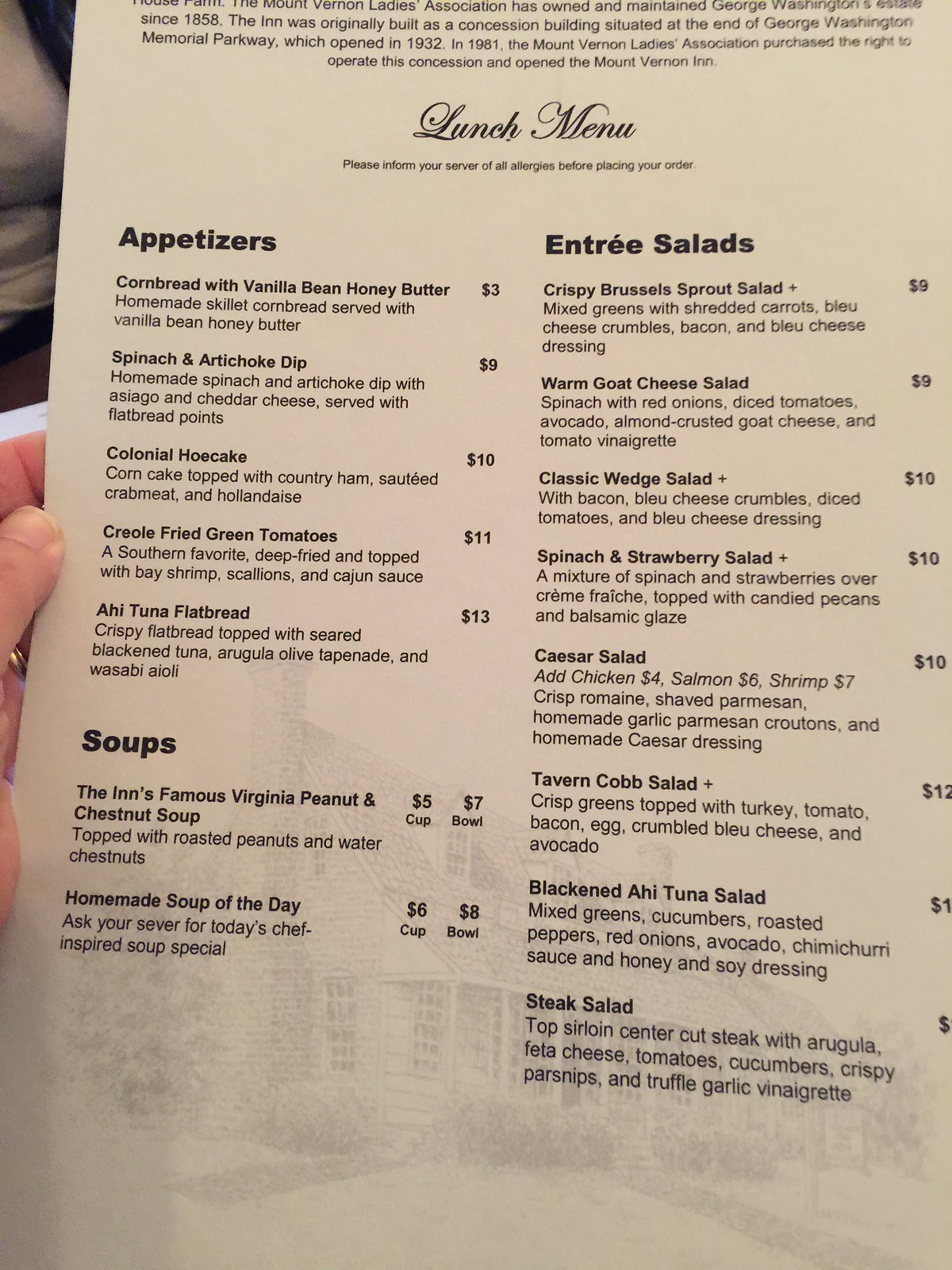A person is holding a lunch menu, which occupies almost the entire frame of the image. Their hand is slightly visible mid-left of the frame, showing part of the palm and the knuckle of the thumb, along with the thumbnail. Just above the thumb, the tip of the pointer finger peeks out from behind the menu. Additionally, the top left corner reveals a small portion of a white shirt sleeve. 

The top of the menu features a block of text detailing the history of the building. Beneath this historical paragraph, the words "Lunch Menu" are elegantly written in black cursive. Following this title, there's a section of small black text that's too blurry to read. 

The menu is organized into two main columns, left and right. In bold black letters, the left column starts with "Appetizers," listing five different appetizers, each with a description and corresponding price. 

Below the appetizer section is "Soups," also in bold, where two kinds of soup are listed. Each soup option includes two sizes: cup and bowl, each with its price noted to the right. 

Further down the left column is "Entree Salads," prominently displayed in bold. This section lists eight different salads, each with detailed descriptions and prices aligned to the right side of the menu.